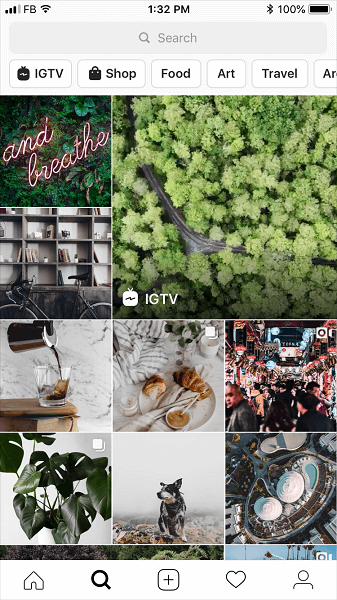In this image, you see a screenshot of a mobile device interface, displaying various status icons and navigation options. 

At the very top of the screen, the status bar indicates the following:
- On the top left, there are three out of four bars of network signal strength, with the network provider labeled as "FB."
- Next to it, the Wi-Fi signal strength is at full, showing three out of three bars.
- The current time displayed is 1:32 PM.
- On the top right, there is a Bluetooth icon, and the battery level is at a full 100%.

Below the status bar, a search field is prominently featured, accompanied by icons for IGTV and Shop. Additionally, there are visible categories like Food, Art, and Travel. The interface displays thumbnails representing these categories, which include images of trees, various food items, and a dog.

At the bottom of the screen, the navigation bar contains several buttons:
- A Home button for returning to the main feed.
- A Search button for finding content.
- An Add button for posting new content.

The image encapsulates a typical user interface of a mobile application, providing a snapshot of the device's status and navigating options at that particular moment.